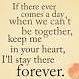This is a very small, low-resolution, square image resembling the style often seen in social media posts, particularly fitting for an older woman's Facebook feed. The background is a creamy beige yellow color with slightly pixelated black text. The text reads: "If there ever comes a day when we can't be together, keep me in your heart. I'll stay there forever." The formatting of the text is irregular, with noticeable indents after certain lines. Notably, the word "forever" stands out at the bottom in a larger, darker, and thicker font, making it more prominent. In the bottom right corner, there's a peach and pink colored heart adding a gentle decorative element. This combination of sentimental text and visual design creates an inspirational quote graphic, reminiscent of a heartfelt message on a sticky note.